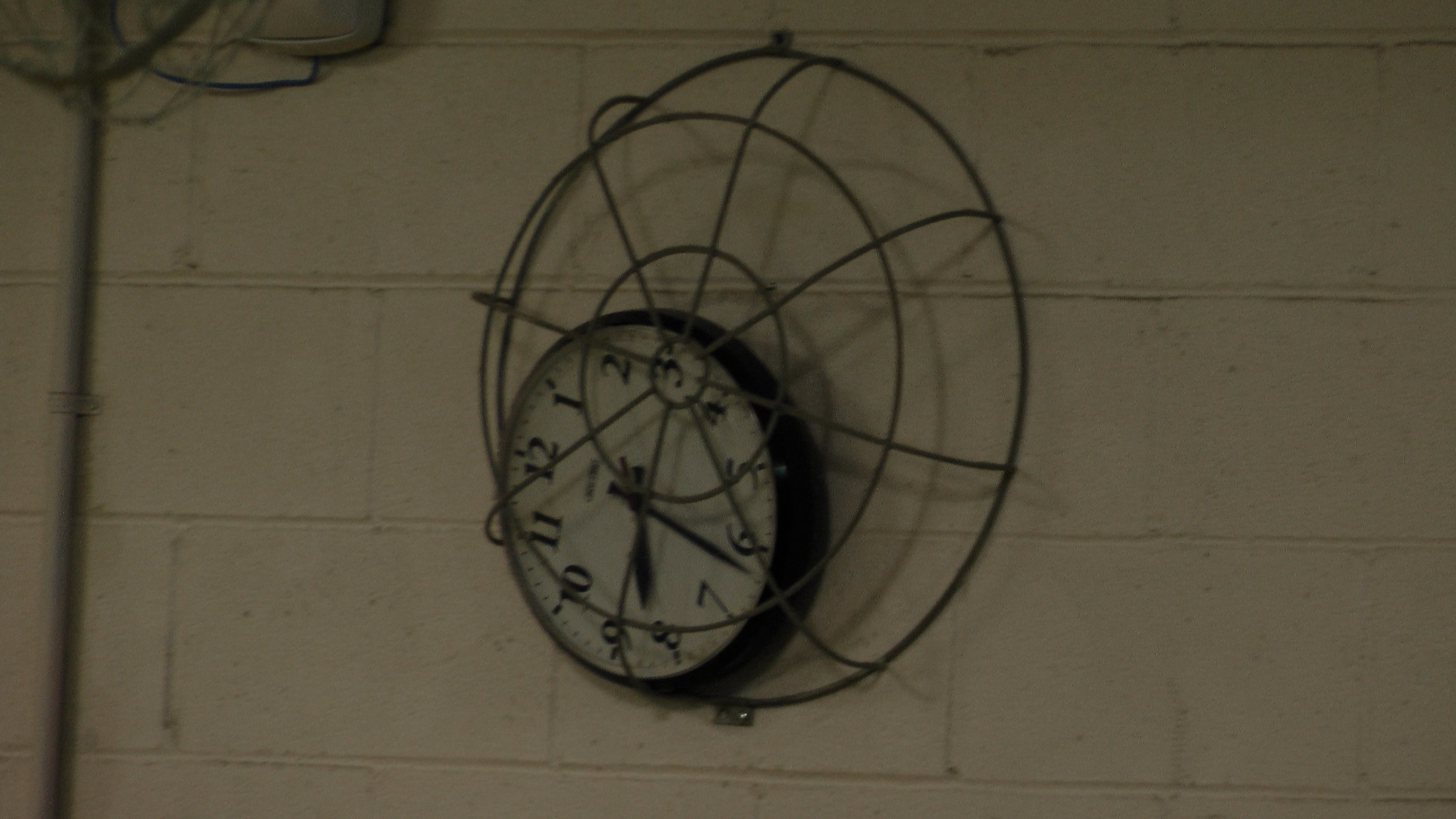This image features a clock that appears to have fallen from its original position but remains suspended against a white brick wall. The clock is contained within a metal bracket, preventing it from hitting the floor and causing potential damage. The clock face displays numbers from 1 through 12, and it has two black hands: a shorter one indicating the hours and a longer one for the minutes. In the upper left-hand corner of the image, there are visible cords and what seems to be an alarm or a large doorbell box. The overall scene captures a moment of disruption while showcasing the sturdy brick wall in the background.